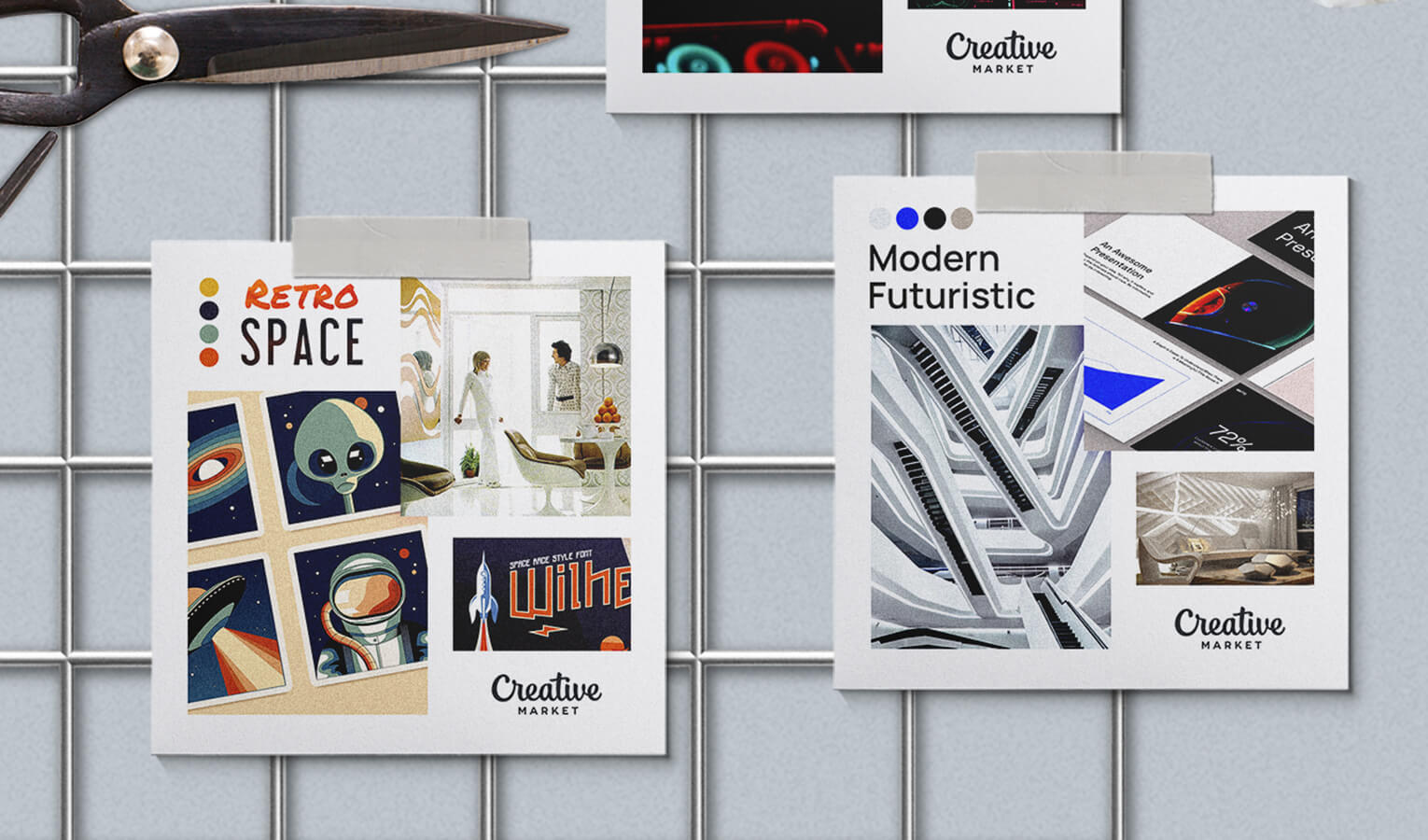This detailed, up-close photo showcases a collection of vinyl art sheets displayed on a light gray metal grate. There are two main posters taped onto the grate. The poster on the left, labeled "Retro Space," features various retro-themed illustrations including a yellow alien, a planet with Saturn rings, a UFO beaming up a light, and an astronaut with a covered visor. There are four color circles in yellow, bluish cyan, and red in the top left corner, and a small image of a couple enjoying themselves in a modern setting is in the top right corner. The words "Creative Market" are printed in the bottom right corner twice, along with a small picture of a room containing modern furniture.

The second poster on the right is titled "Modern Futuristic" and showcases gray, blue, black, and green color circles. Additionally, there is an image of escalators moving in all directions and a picture insert of a room's interior that is partially obscured. The bottom of this poster also reads "Creative Market." Overall, the scene is set against a light gray background with a pair of pewter-colored metal scissors visible in the upper left corner.